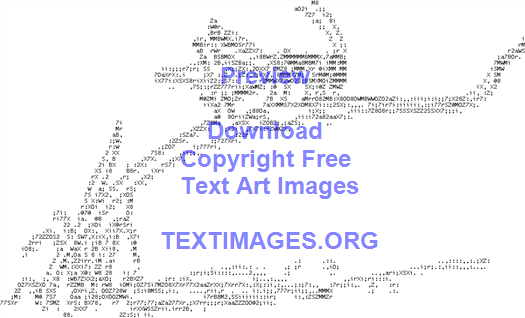This image is a detailed piece of ASCII art, a form of text art created using keyboard symbols, including punctuation, letters, and numbers, all rendered in tiny black characters on a stark white background. The artwork depicts a scene of nature featuring a long blade of grass, which starts in the bottom left corner, curves gently upwards, plateaus slightly, then ascends again before curving into a twirl at the top right corner. Below this blade of grass, there's an area that represents the ground. Intricately nestled on the middle section of the blade is a detailed depiction of a grasshopper, identifiable by its two antennas, long back legs, and shorter front legs. Above the image, in semi-transparent purple font, the text reads: "Preview download copyright-free text art images textimages.org". This text not only labels the artwork but suggests a source and repository for similar ASCII art, reflecting a nod to the early days of computing in the 1980s. This blend of textual art and informative text creates both a visually striking and educational piece.